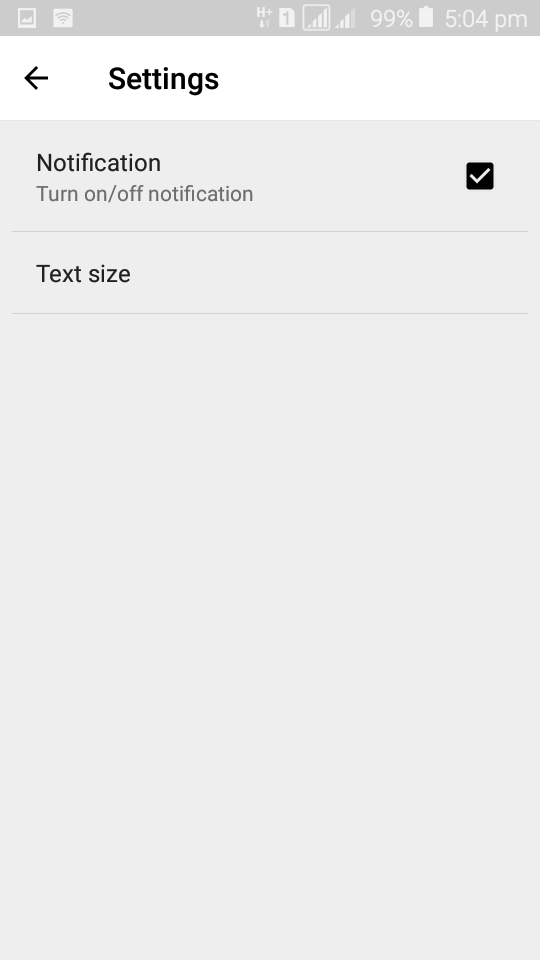The image is a screenshot taken from an Android phone, displaying a specific settings page. In the top right corner, the time is shown as 5:04 PM, and the battery charge indicator is at 99%. In the top left corner, the title "Settings" is visible, accompanied by a left-pointing arrow, which functions as a back button.

Below the title, there are two selectable options. The first option is labeled "Notifications," with a small checkmarked box to its right. The checkmark inside the box is white, while the outline of the checkbox is black. The second option listed is "Text size." The page features a predominantly white to gray background. The screenshot effectively captures the details and layout of the settings page on the Android device.